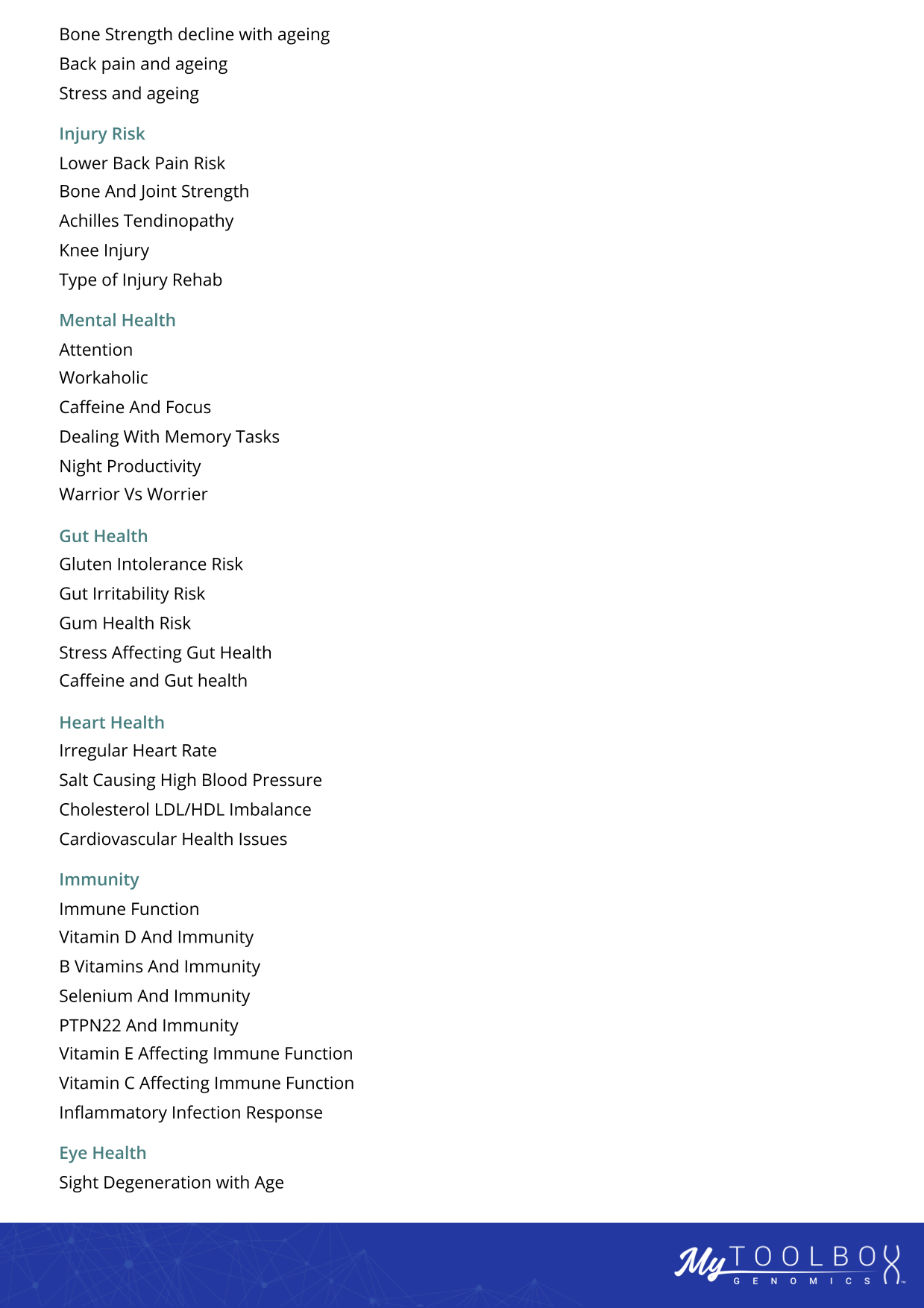A screenshot taken from a mobile device screen shows a health-related application interface. On the left side of the screen, there is a vertical list of health categories displayed in bold black and blue text. At the top, under the section likely labeled "Bone or Skeletal Health," there are entries such as "Bone Strength Decline with Aging," "Back Pain and Aging," and "Stress and Aging." This is followed by the "Injury Risk" category, which includes entries like "Low Back Pain Risk," "Bone and Joint Strength," "Achilles Tendinopathy," "Knee Injury," and "Type of Injury Rehab." The "Mental Health" category features topics such as "Attention," "Workaholic," "Caffeine and Focus," "Dealing with Memory Tasks," "Night Productivity," and "Warrior vs. Worrier."

The right side of the screen is entirely blank and white. At the bottom of the screen, there is a rectangular button stretching across the entire width of the device, labeled "My Toolbox." The word "My" is in cursive, while "Toolbox" is in regular font with the "X" noticeably larger and curved. Other categories visible further down the list include "Gut Health," "Heart Health," "Immunity," and "Eye Health," each with their own subtopics.